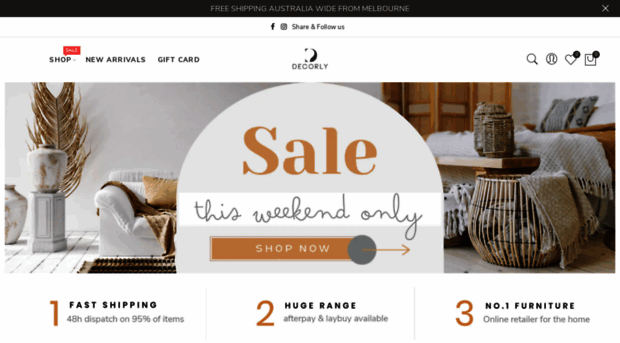The screenshot captures a webpage with a landscape orientation, approximately twice as wide as it is tall. At the very top, the page features a thin black bar spanning horizontally, occupying about 5-10% of the screen's height. Centered within this black bar is bold, white text reading, "Free Shipping, Australia Wide from Melbourne." 

Below the black bar is a section with a white background. This section includes icons for social media, alongside the words "Share" and "Follow Us." Proceeding further down, on the left side of the screen, slightly indented, are three menu options: "Shop," "New Arrivals," and "Gift Card." Above the "Shop" menu, in the upper right corner, there is a red rectangle with the word "Sale" inside it.

Centered horizontally across the page, adjacent to the menus, the text "Deckerly" is prominently displayed. To the far right, a series of icons are aligned: a magnifying glass (likely representing search), an empty profile picture, a heart (possibly for favorites), and an envelope.

Dominating the main content area is a primary banner. This banner showcases a room bathed in white, including a white floor and a white backdrop wall. A white couch is positioned centrally, accompanied by a table to the right, draped with a white blanket. Centrally overlaid on this serene scene is the word "Sale" rendered in a tan color.